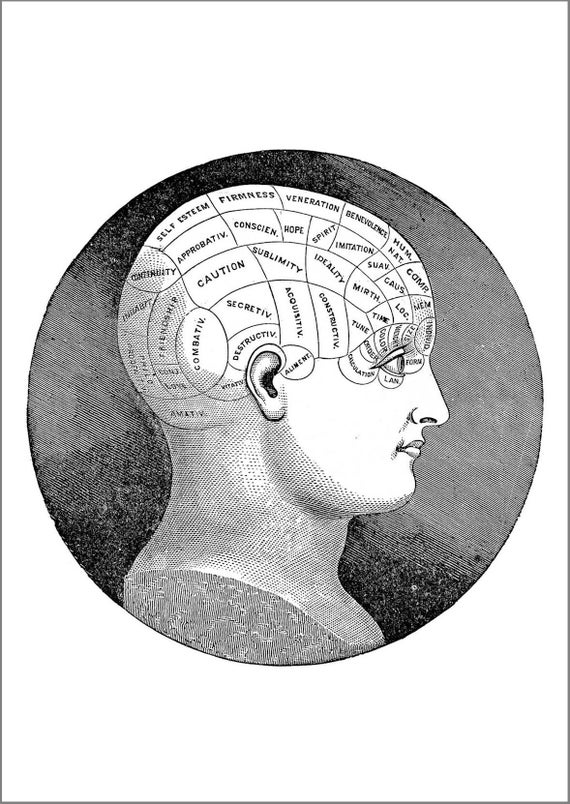This black and white illustration features a bald human head presented in a classic phrenological diagram style, framed by a black border. The head-and-shoulders bust is set against a black and gray shaded circular background. The head is oriented to the right, allowing visibility of the side profile, which includes one eye, the nose, lips, and a single ear. The upper portions of the head are sectioned into numerous labeled areas, each representing different supposed faculties and traits of the brain as per phrenological belief. Some of the identifiable labels include self-esteem, firmness, veneration, benevolence, caution, sublimity, ideality, spirit, imitation, conscience, and acquisitive, among others. The meticulous detailing of the head's regions underscores the period's attempt to map personality and character traits onto specific physical areas of the brain.